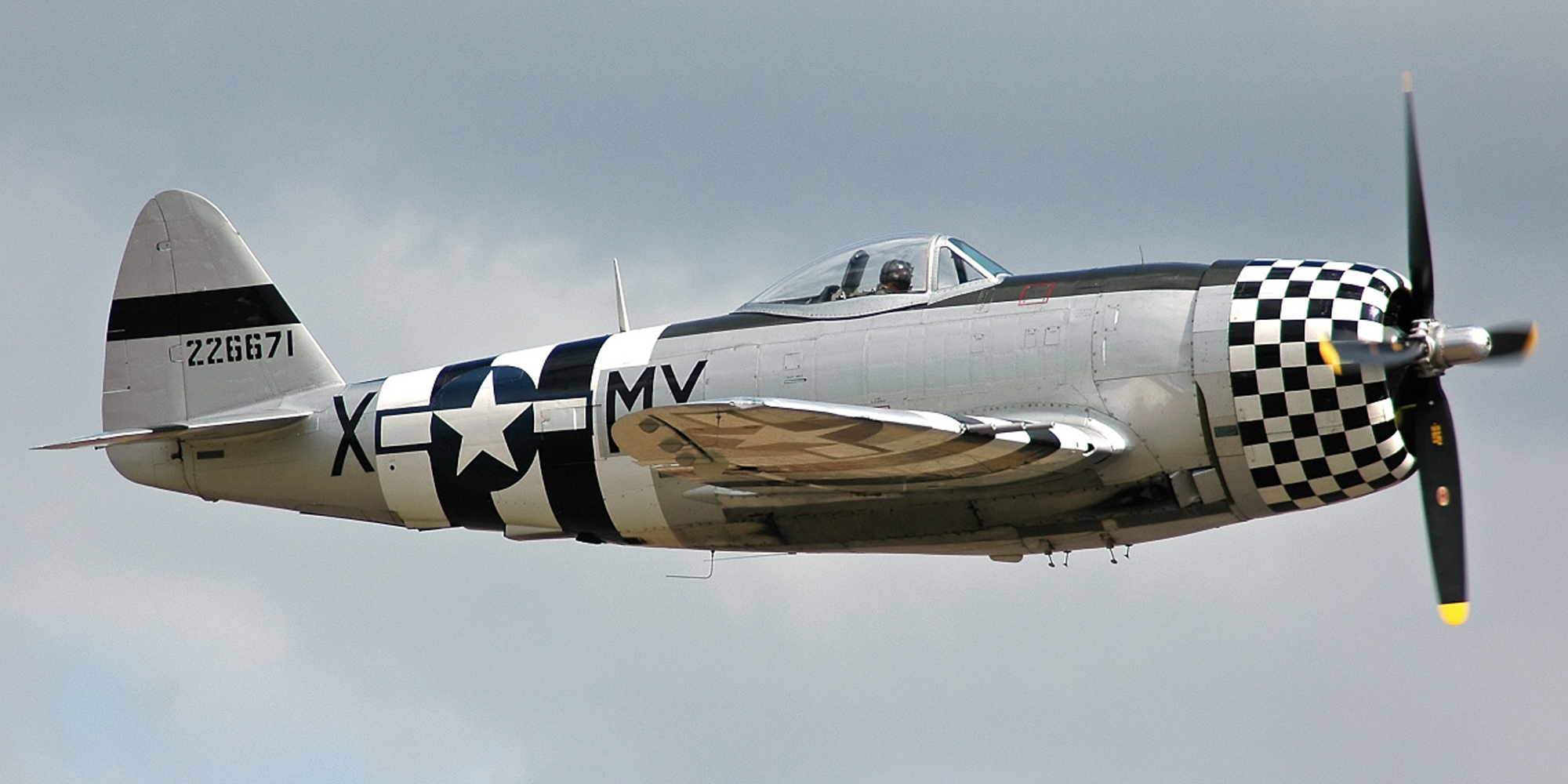This image captures a vintage World War II-era warplane prominently positioned in the center of a horizontally rectangular frame against a clear blue sky dotted with faint white clouds. The aircraft boasts a sleek silver-gray metallic body. Most strikingly, its nose features a distinctive black and white checkered pattern, while the propellers, which number three, are depicted in black with yellow tips, poised for flight.

The tail of the aircraft, shaped like a slightly curved triangle, exhibits an eye-catching design with alternating strips of blue and white, complemented by a bold white star set against a blue circle. Below this emblem, the identification number 226671 is clearly visible. Markings on the side include the letters X, M, and what appears to be either a Y or V.

The canopy, with its clear glass window, reveals the figure of the pilot, identifiable by the black helmet. This historical plane's meticulously detailed features make it a compelling subject against the serene azure backdrop.